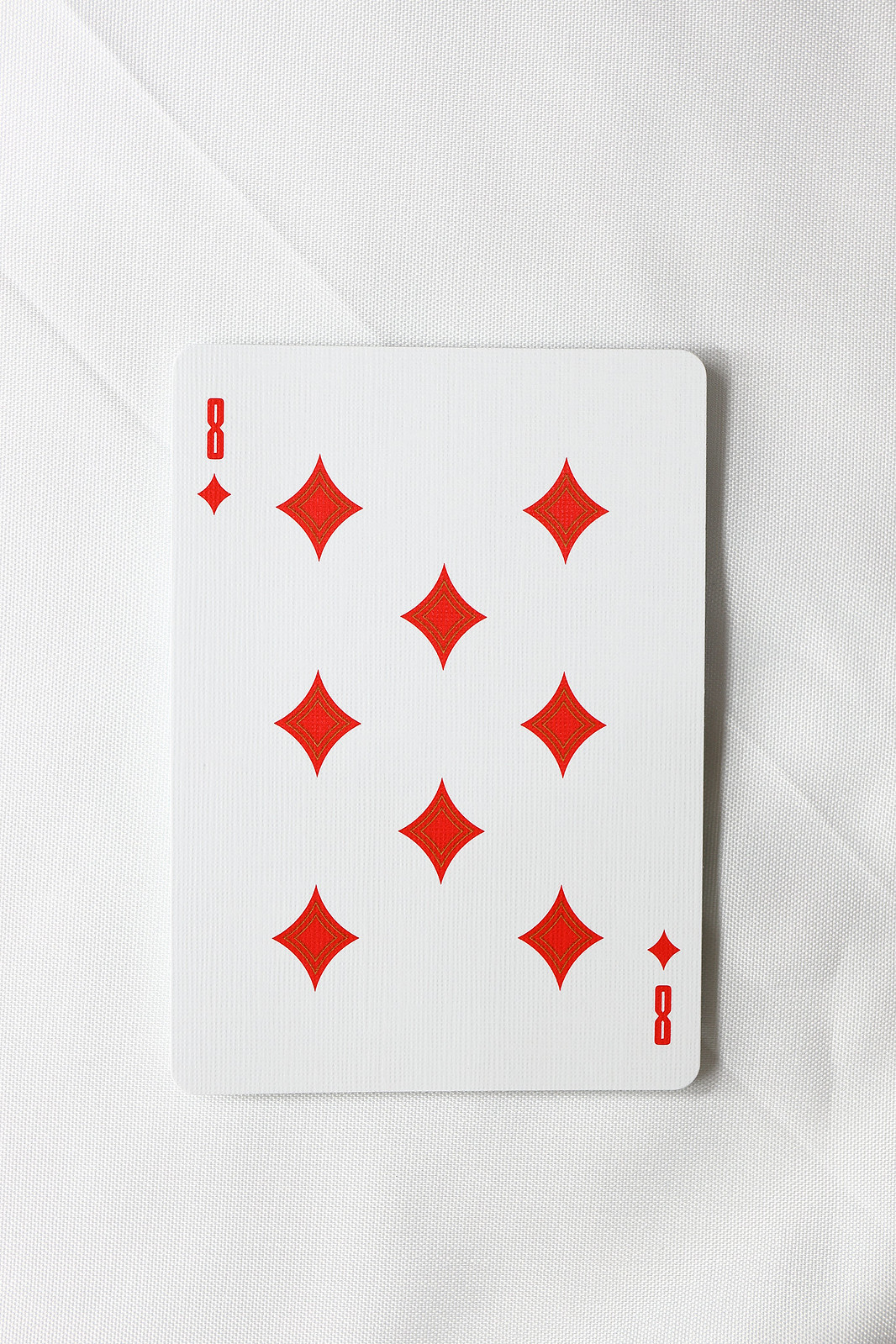A detailed image depicts an Eight of Diamonds playing card set against an all-white background. The backdrop features a subtle diagonal stripe extending from the bottom left corner to slightly above the top right corner, discernible by its slightly different hue of white. The playing card itself is also white, small, and rectangular, casting a delicate shadow along its right edge. Both the top-left and bottom-right corners of the card display the number "8" and a four-pointed diamond symbol beneath it. Centrally, eight diamond shapes are artfully arranged in a symmetrical pattern: two diamonds at the top, followed by a set of three diamonds forming a triangle, another set of three diamonds creating a similar formation beneath, and finally, two more diamonds at the bottom.